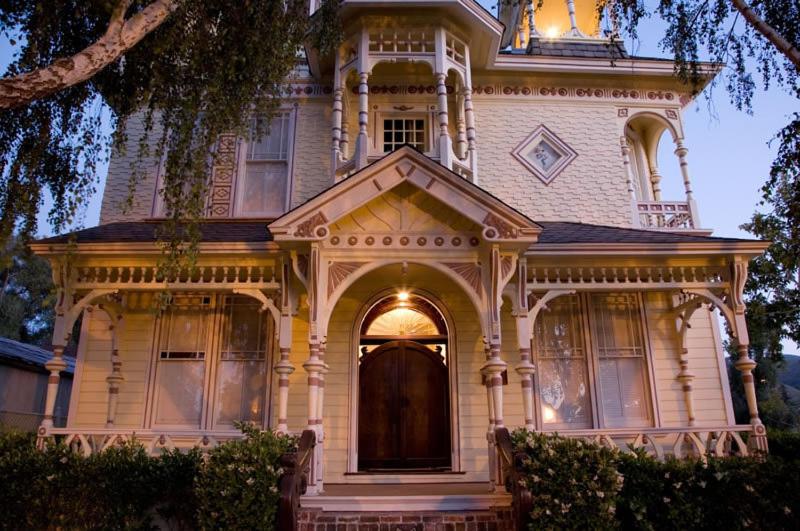This photograph showcases a large, beautiful house that appears to be either colonial or plantation-style architecture, possibly located in the southern United States, such as in Georgia or South Carolina. The house is white with textured siding and features a prominent porch area adorned with lattice and small white pillars. The front entrance, accessible via steps bordered by red and gray bricks, has an arched brown door surrounded by railings and illuminated by a glowing light above. The second floor boasts a balcony supported by four pillars. The exterior is complemented by lush foliage, including bushes with small white flowers and a striking tree with hanging leaves resembling a weeping willow or wisteria, cascading in front of an upstairs window. The elegant dwelling's classical frontage, surrounded by verdant shrubbery and illuminated by soft light, conveys a serene and picturesque setting.